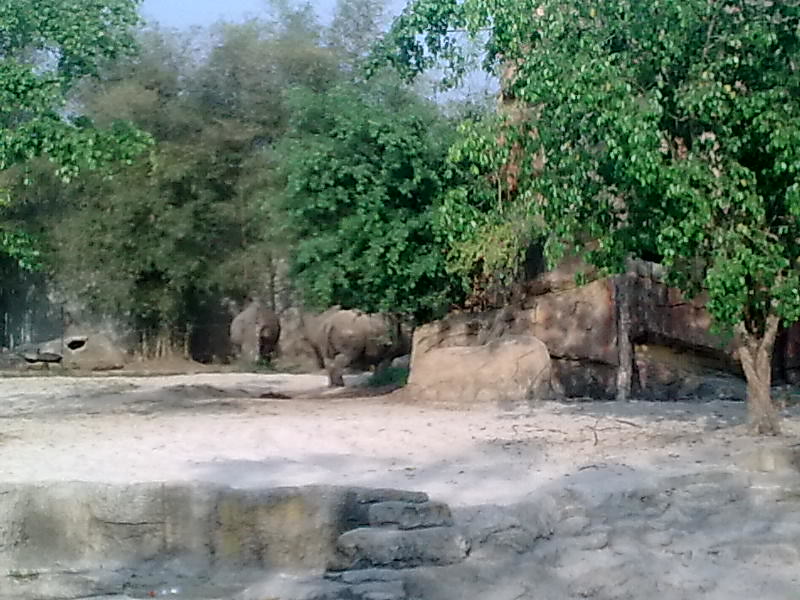This daytime color photograph appears to be taken outdoors within a zoo setting. Dominated by a variety of green trees, both natural and possibly artificial, the scene also contains several sandy and dry areas with shallow, stacked rock walls that contribute to an artificial habitat, commonly seen in zoos. Towards the left-center of the frame, you can discern the blurry and indistinct backsides of large animals, likely elephants, though they could also be rhinoceroses or hippopotamuses, given the lack of clear detail. There are no other people or animals visible in the scene, which is under a bright, cloudless sky. The overall palette of the image includes shades of green from the trees, browns and grays from the rock formations, and vibrant sky blue, lending to a tranquil but somewhat arid atmosphere.